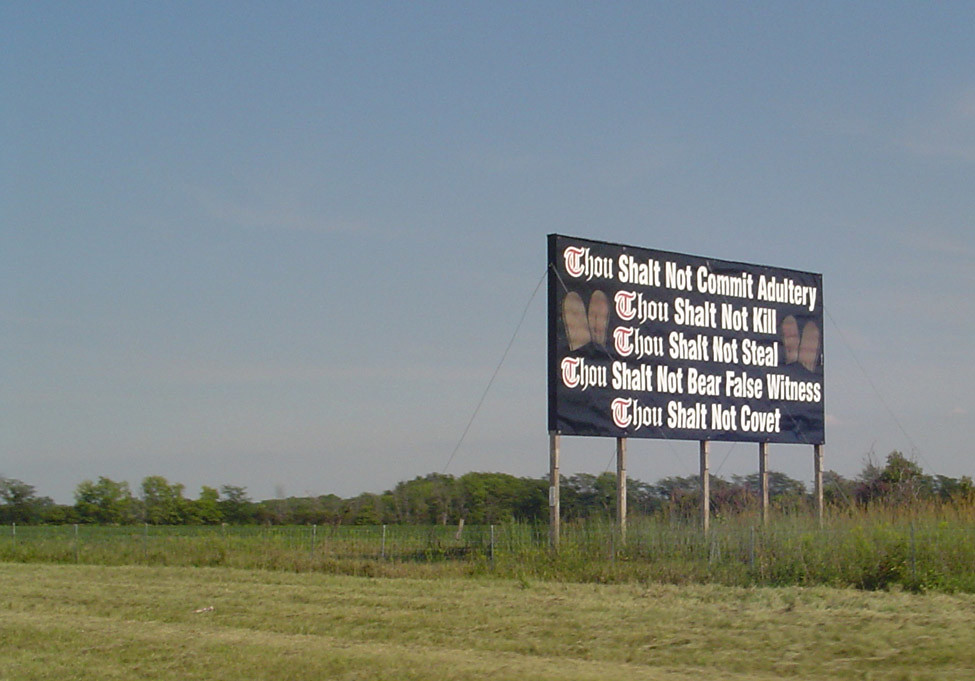A large, horizontal billboard stands prominently in a grassy field, likely positioned to be visible from a nearby road. The backdrop of the scene includes a light blue sky, a distant horizon adorned with various trees, green scrub grass, and sections of mown grass. A metal post and wire fence runs through the landscape, adding to the rural ambiance. The billboard itself is supported by five sturdy wooden posts and features a dark background, possibly black or dark blue. Displayed in five distinct lines, the text on the billboard reads: "Thou shalt not commit adultery," "Thou shalt not kill," "Thou shalt not steal," "Thou shalt not bear false witness," and "Thou shalt not covet" — all of which are commandments from the Biblical Ten Commandments.